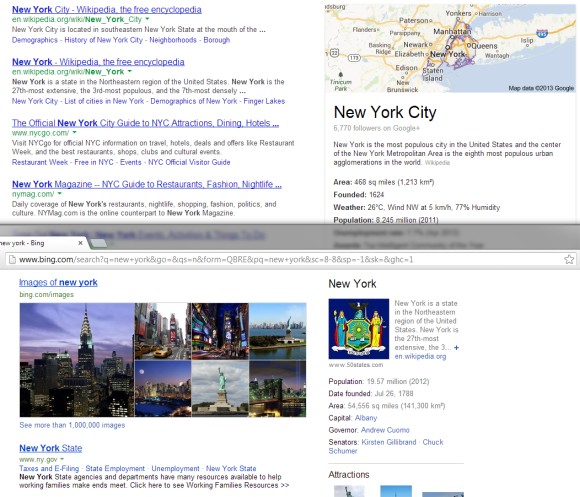The image is divided into two distinct sections. The top half displays a screenshot from Google Maps showcasing the New York metropolitan area. Prominently featured on the map are several key locations including New York, Queens, Yonkers, Paterson, Newark, Elizabeth, Edison, and Flanders. The map’s right side highlights two large bodies of water in a light blue hue. In the upper left corner of this section, multiple hyperlinks in blue text are visible, reading: "New York City," "New York," "The Official New York City Guide," and "New York Magazine."

The bottom half of the image is a screenshot from the Bing website, evident from the URL "bing.com" located at the top left. This section also centers on New York, with a smaller boxed image positioned at the top right corner that shows two individuals. Beneath this image, several data points are listed: Population (19.57 million), Date Founded, and Area Capital, providing detailed information about New York.